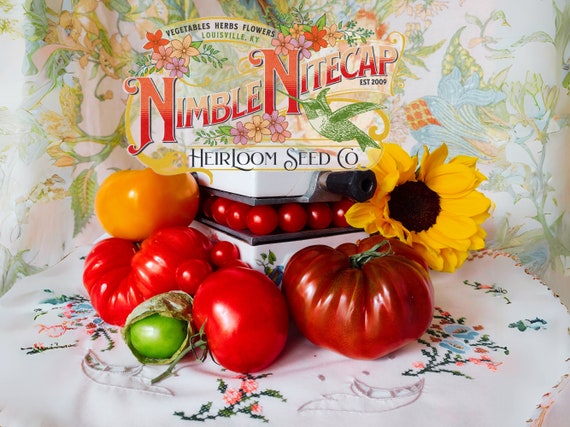This advertisement for Nimble Nightcap Heirloom Seed Company, established in 2009 and based in Louisville, Kentucky, creatively displays an assortment of heirloom tomatoes arranged centrally on a table. The tomatoes exhibit a vibrant color spectrum ranging from dark red, bright red, and orange to green, yellow, and even rare hues like black and white. Nestled among the tomatoes on the right side is a decorative fake sunflower with yellow petals and a dark center. All of these elements rest on a charming white doily, reminiscent of hand-stitched designs found in a grandmother’s home, adding a nostalgic touch to the setup. 

Above the table, the company's logo and name “Nimble Nightcap” is prominently displayed in bright reddish-orange letters, with additional text in black lettering, including "Vegetable, Herbs, Flowers, Louisville, Kentucky" and "Heirloom Seed Company." The backdrop of this visually appealing setup is a floral-patterned curtain or wallpaper featuring pastel colors in blues and greens, complete with various flower heads in orange and other hues. This harmonious combination of heirloom vegetables and decorative elements effectively promotes the company's traditional and artisanal seed offerings.